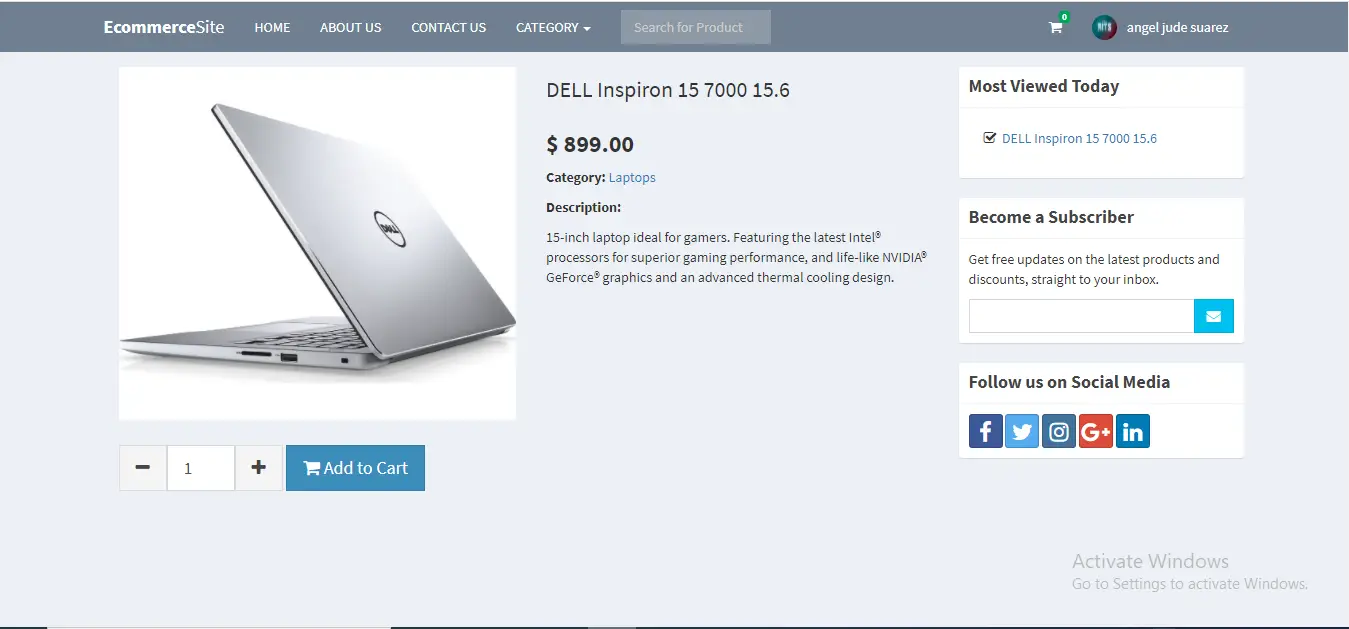Screenshot of an e-commerce website displaying a silver Dell Inspiron 15 7000 series laptop for sale. The website's top bar is gray, containing menu options labeled "E-commerce Site," "Home," "About Us," "Contact Us," and "Category," alongside a search bar with the placeholder text "Search for product." A shopping cart icon and the name "Angel Ju Suarez" suggest that a user is currently logged in.

The main content features a partially open Dell laptop, showcasing its silver exterior and the distinctive round Dell logo centered on the back. The visible portion of the keyboard hints at the laptop's sleek and modern design. Below the image, the laptop is identified as a Dell Inspiron 15 7000 15.6", priced at $899.

Categorized under "Laptops," the product description highlights its suitability for gamers, boasting the latest Intel processor, lifelike NVIDIA GeForce graphics, and an advanced thermal cooling design for optimized performance. Additional website features seen in the screenshot include options to view the "Most Viewed Today" products and an invitation to "Become a Subscriber."